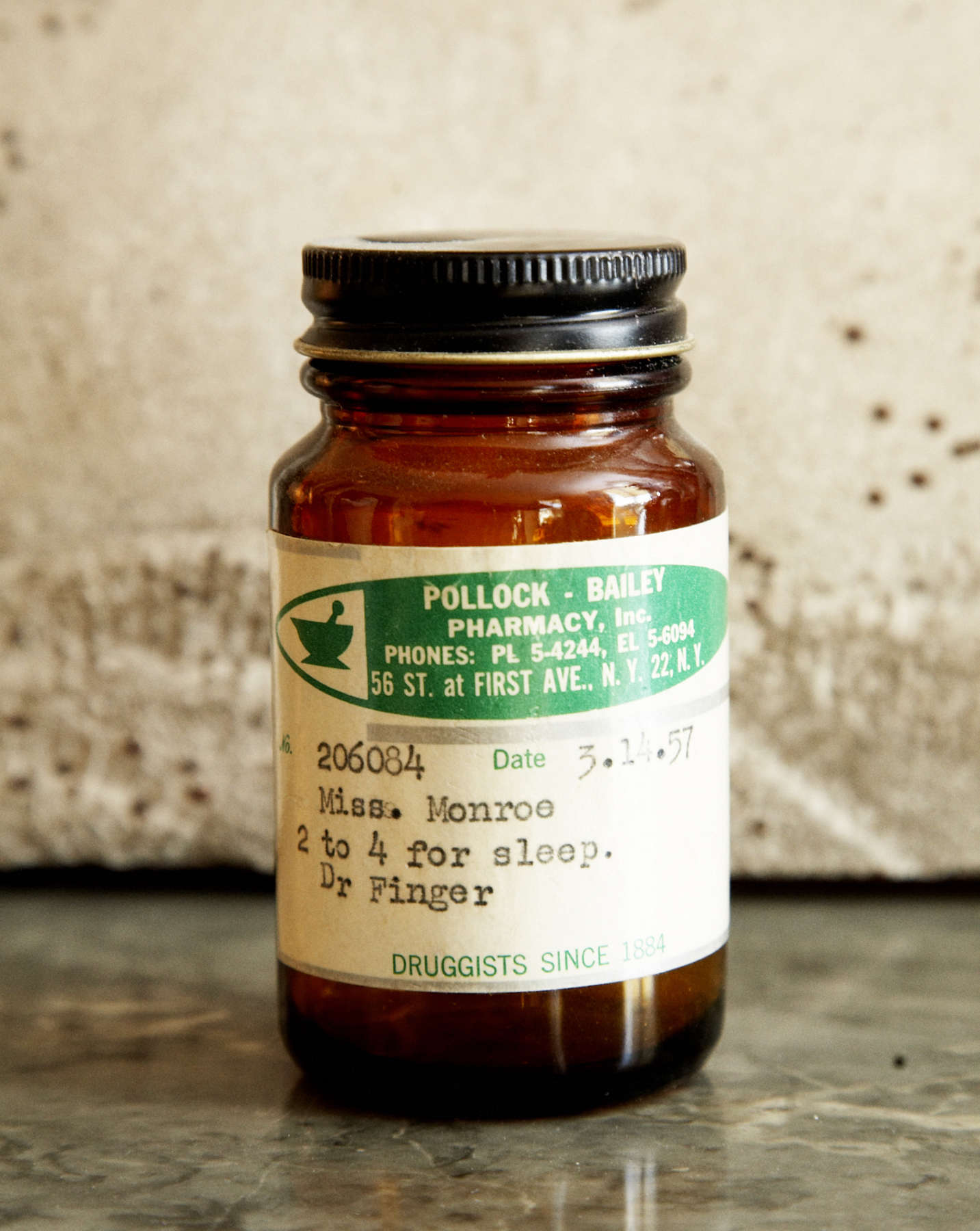This photograph captures an antique prescription bottle displayed on a gray marble surface with a cream-colored wall in the background. The bottle itself is made of brown glass and is topped with a black, screw-on metal cap. A white label encircles the middle of the bottle, prominently featuring a green oval with white lettering that reads "Pollock Bailey Pharmacy, Inc." Inside the oval, there's also an illustration of a small bowl with a pulverizer stone. The label includes the pharmacy’s phone numbers, PL 5-4244 and EL 5-6094, and its address at 56th Street and First Avenue, New York, 22, New York.

The rest of the white label is detailed with black lettering, citing the prescription number, 206084, and the date, 3-14-1957. The patient's name, "Ms. Monroe," and the dosage instructions, "2-4 for Sleep," are also clearly printed. The prescribing doctor is identified as Dr. Finger. Additionally, in green lettering at the bottom of the label, it states "Drug Assist since 1884." This vintage medicine bottle is not only a piece of medical history but also a glimpse into pharmaceutical practices from the mid-20th century.